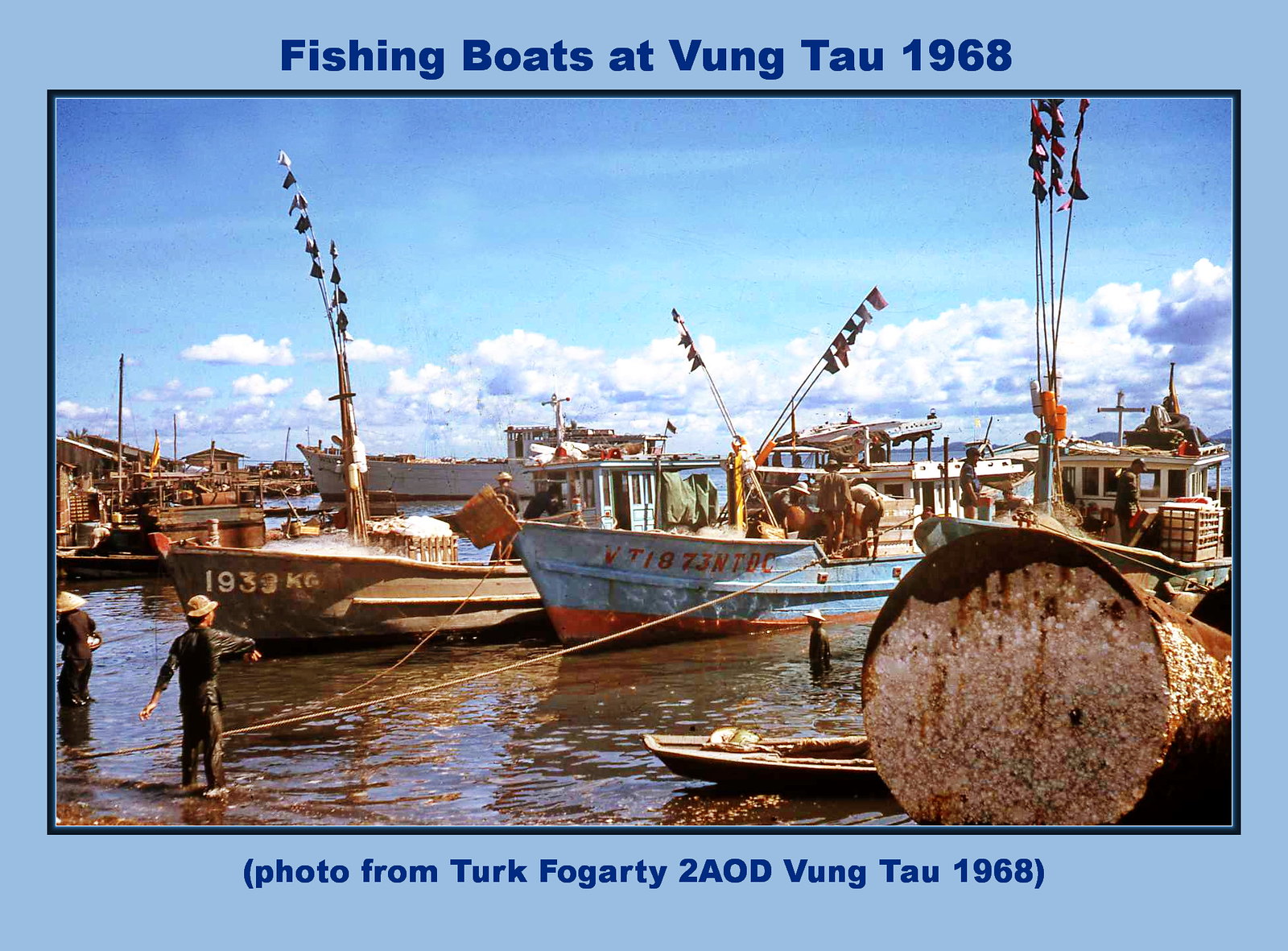The image is a vibrant, full-color photograph of fishing boats at Vung Tau in 1968, as indicated by the text in dark blue ink against a light blue border at the top. It also details that the photo was a gift from Turk Fogarty to AOD Vung Tau, 1968, noted at the bottom. The scene features shallow waters near a dock under a mostly sunny sky with white fluffy clouds. Dominated by a central blue fishing boat with an orange hull and white cabin, the image showcases two Vietnamese men to the left engaging with people on the boat. This boat is flanked by two others, with the one on the left marked "193 KG". Ropes connect the boats to the shore, emphasizing their proximity to land. Adding to the intricate details, the lower right-hand corner displays a large drainage pipe and a smaller canoe-like boat. The borders of the photograph are also notable, with an outer light blue frame and a thinner black inner border, framing the entire picturesque setting with precision. The photograph almost has the clarity and detail of a drawing, capturing a snapshot of a historical and cultural moment.